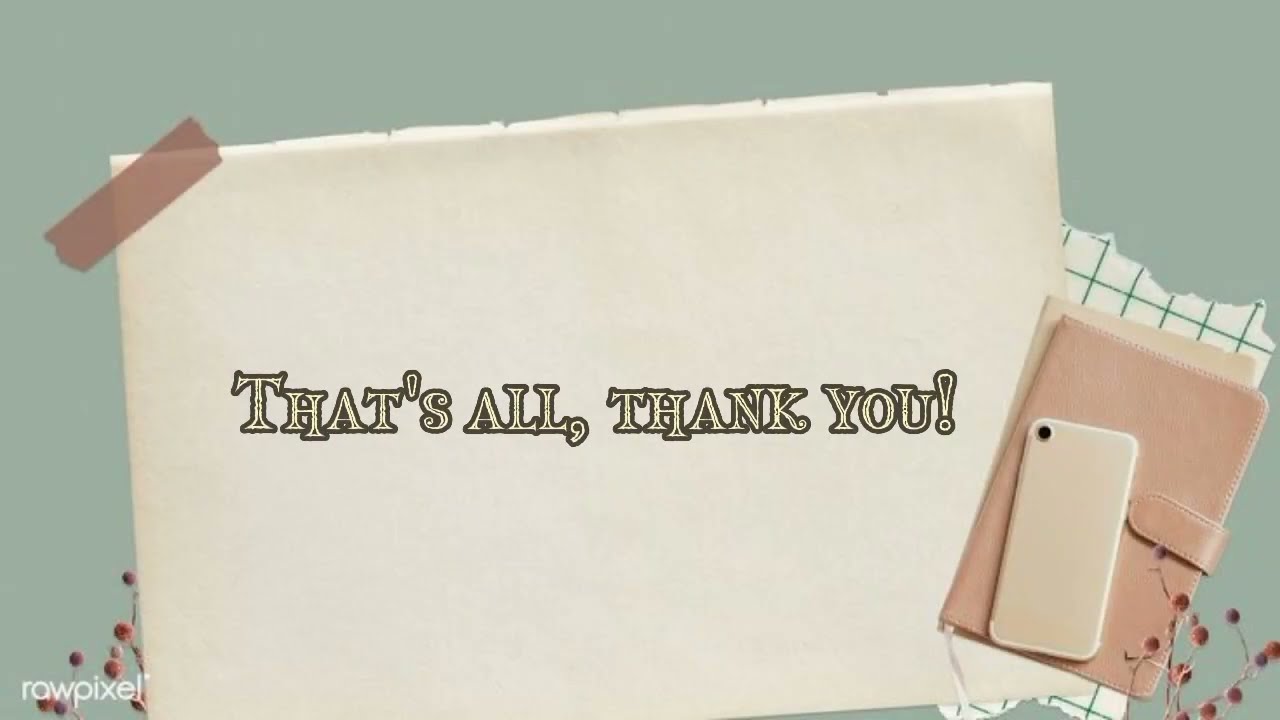The image features a creatively designed "THAT'S ALL, THANK YOU!" message in bold, black-outlined, off-white capital letters with an exclamation point, centered on a piece of white paper that appears ripped at the top. This paper is taped to a background, possibly a sage-green or light blue surface, with partially transparent brown or pale pinkish tape at the corners. In the bottom right corner of the image lies a white smartphone, back facing up, resting on a leather-bound, pink or soft peach-colored journal with a strap closure. Below this journal is an off-white card and a torn piece of graph paper. Decorative elements include small brown branches adorned with mauve, reddish berries positioned at both the bottom left and right corners. The entire setup is framed against a dark turquoise background, and the subtle text "raw pixel" is visible in the bottom left corner.